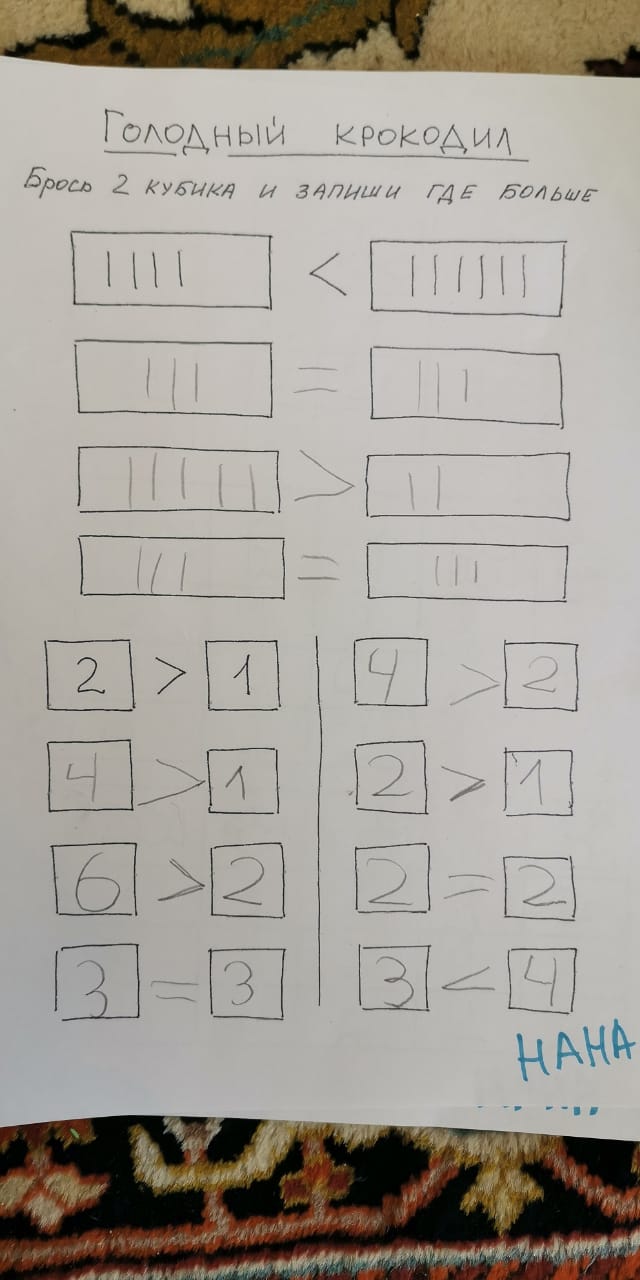In the photograph, a rug featuring an intricate black, yellow, and white pattern with various lines and designs forms the background. Lying atop the rug is a white piece of paper covered in black writing. The writing appears to be in a different language, possibly Russian, indicated by the unfamiliar alphabet. At the top of the paper, there is a section of underlined text. The layout of the document includes several geometric shapes: boxes, triangles, and equal signs. Specifically, there are triangles positioned between some of the boxes towards the top, and equal signs connecting other boxes. Below these, there are rows of boxes filled with different numbers, some accompanied by arrows or equal signs. In the bottom right-hand corner of the page, the word "HAHA" is written in blue ink.